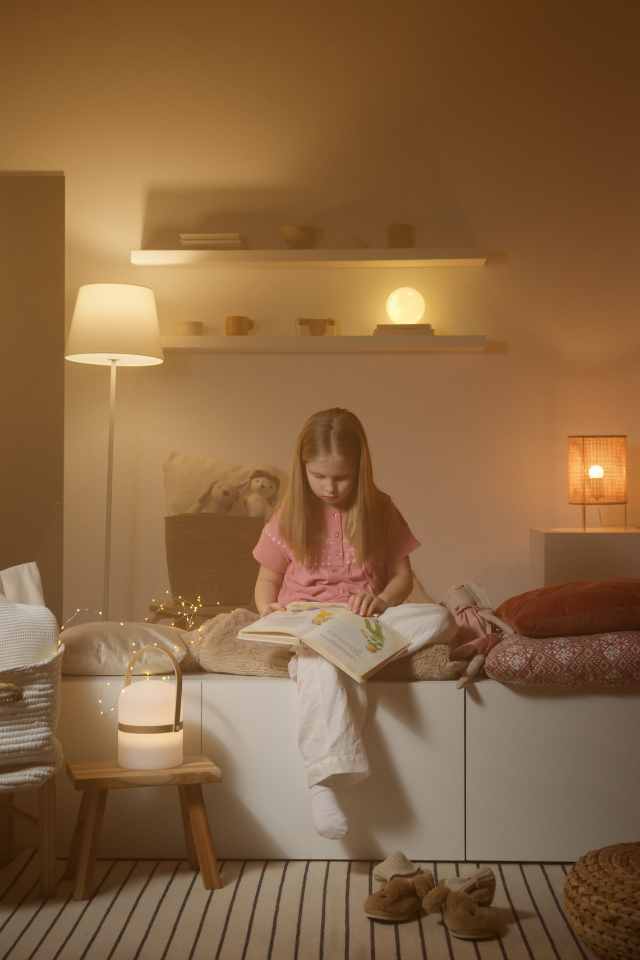The image is a color photograph in portrait orientation, capturing a cozy living space in a representational realism style. The focal point is a young girl, approximately eight years old, with long blonde hair. She is sitting on a low-profile white sofa, intently reading a book in her lap while facing downward. She wears a pink pajama top, cream-colored pajama pants, and white socks. The sofa serves as her comfortable reading nook, adorned with an assortment of pillows in beige and dark red hues.

In front of her, the beige wooden plank floor features a pair of brown leather boots and a pair of slippers. To her left sits a small wooden stepstool, upon which rests a glowing lantern, creating a warm, inviting ambiance. The wall behind the girl is light beige and holds two floating white wooden shelves. These shelves display various objects, including a round moon-like light and other small decorative items.

Further in the background, a tall floor lamp with a white shade stands next to a doorway, complementing the room's soft lighting. Completing the scene, a subtle presence of nature-inspired decor is evident with string lights mimicking lightning bugs draping around the room, adding a whimsical touch to this serene reading environment.